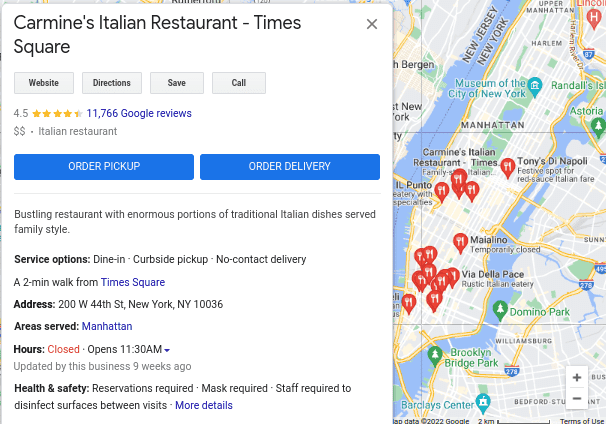Carmen's Theme Italian Restaurant, nestled in the heart of Times Square, offers a culinary journey through traditional Italian cuisine. It boasts an impressive 4.5 out of 5 star rating on Google, with nearly 12,000 rave reviews. This semi-expensive eatery, indicated by two dollar signs, is well-regarded for its enormous portions served family-style, perfect for sharing.

The restaurant provides multiple service options including dine-in, and both pickup and delivery orders, easily accessible through their website. A quick glance at the map reveals several Carmen's locations dotted throughout Manhattan, with a notable cluster near Lincoln Center and the Museum of the City of New York.

Carmen's Theme is a bustling hub just a two-minute walk from Times Square, located conveniently in Manhattan. The restaurant opens its doors at 11:30 AM and, in light of COVID-19, has implemented health and safety measures such as mandatory masks and thorough disinfection of surfaces between visits.